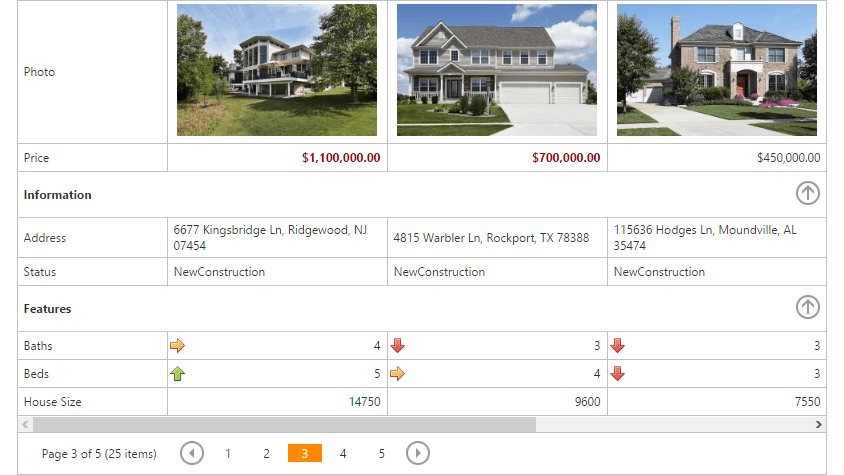This image displays detailed real estate listings for three different houses, each with specified prices, addresses, and property features:

1. The first house is priced at $1.1 million. It is located at 6677 Kingsbridge Lane, Ridgewood, NJ 07454. This new construction boasts five bedrooms and four bathrooms.

2. The second house has a listed price of $700,000. Its address is 815 Wobbler Lane, Rockport, TX 78388. This property features a total of three bedrooms and four bathrooms.

3. The third house is valued at $450,000. It is situated at 1156 Hodges Lane, Moundville, AL 35474. This home includes three bedrooms and three bathrooms.

Each property offers distinctive features and is situated in different regions, catering to various preferences and budgets for potential buyers.